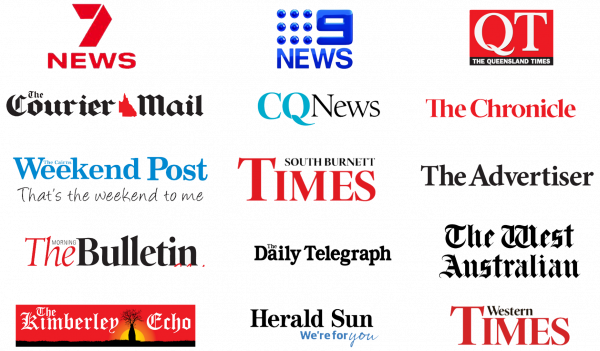In the upper left corner of the image is the number "7" in red text. Directly beneath it, also in red, is the word "NEWS." To the right of this, the text "9 NEWS" is displayed with several dots beside it. Further to the right, there is the name "QT The Queensland Times" followed by "The Courier-Mail," "CQ News," "The Chronicle," and "Weekend Post." Underneath these names is the phrase "The Weekend to Me."

Below this lower section is "South Burnett Times," with "Times" in bold, red, uppercase letters. Over to the right, in black text, is "V Advertiser." Below "V Advertiser," slightly to the left, is "V Bulletin," with the letter "V" highlighted in red. Following this is "Daily Telegraph."

On the lower end of the image, "The West Australian" is shown in a Times New Roman font. In the bottom left corner is "The Kimberley Echo," which features an accompanying graphic of a black, branchy tree. Next, "Herald Sun" is displayed, and underneath it, in blue text, is the phrase "We're For You."

Finally, in the bottom right corner in smaller text, the word "Western" appears, with the term "Times" below it, written in bold red text.